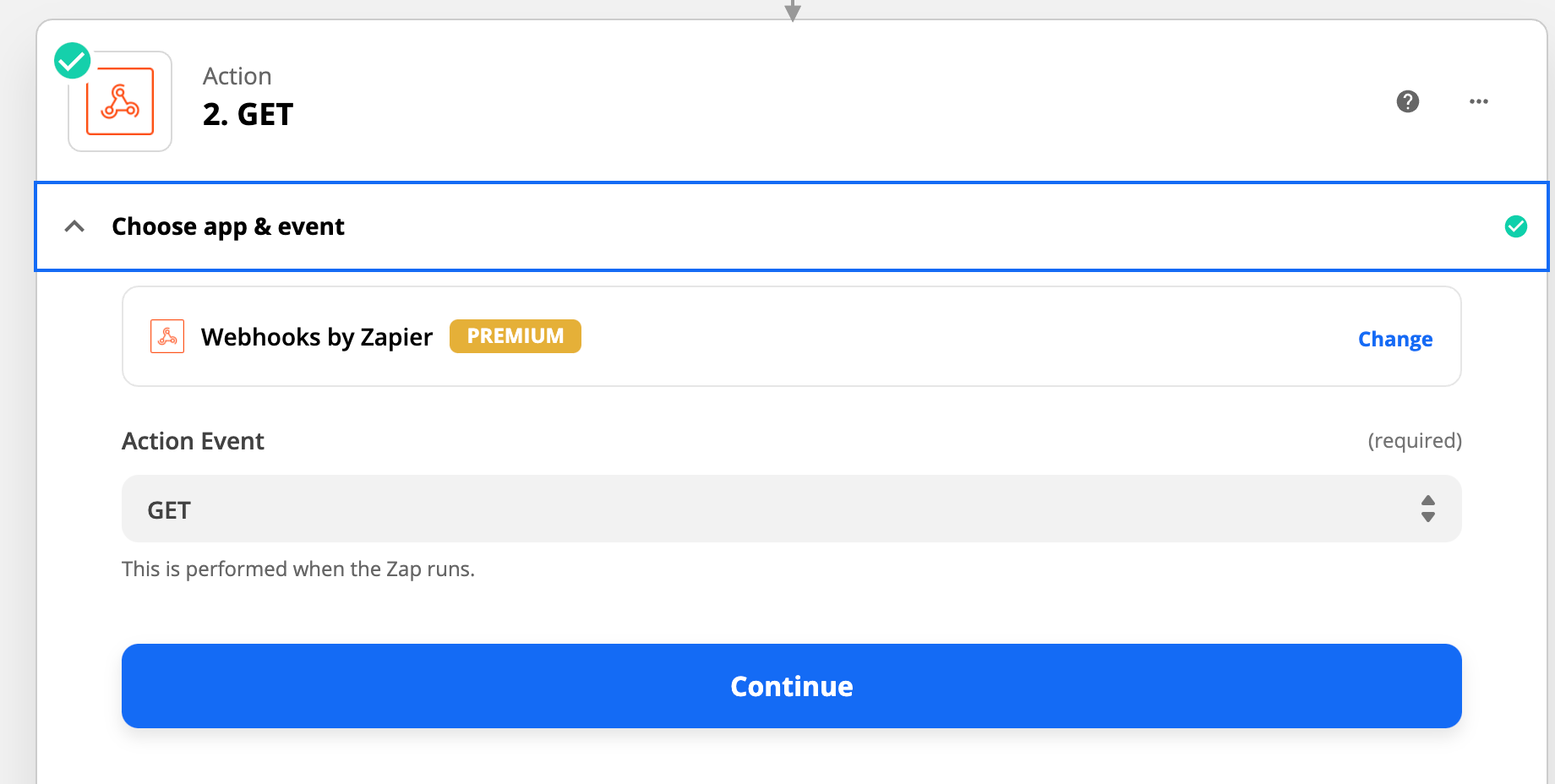The image showcases a section of a web page dedicated to creating and managing web events, specifically using the platform "Zappler." The white background highlights various interactive elements and instructions:

- On the top-left, a green checkmark signifies completion or validation.
- Adjacent to it, there's an orange square emblem with a central orange triangle.
- To the right of these symbols, the text "Action" is displayed in black, followed by "Event: GET" indicating the type of action being defined.
- Beneath this, there's an option labeled "Choose App & Event," highlighted by a black border, with another green checkmark to its right.
- Further down, the label "Webhooks by Zappler" appears, marked as a premium feature in yellow. The word "Change" is clickable and marked in blue.
- Reiterated below this, "Webhooks by Zappler," is shown again with the labels "Action Event: GET" specified for clarity.
- At the bottom of the section, a blue button labeled "Continue" prompts the user to proceed.
- In the top-right corner, there is a gray question mark icon for help and three gray dots for additional settings or actions.
- A downward pointing arrow is centrally located, likely indicating a collapsible or expandable section.
- Finally, at the bottom, a noted statement indicates, "This is performed when Zapp runs," clarifying the sequence of actions.

This detailed layout illustrates the configuration interface for setting up a specific web action using Zappler's services, ensuring users can easily navigate and complete their desired tasks within the platform.